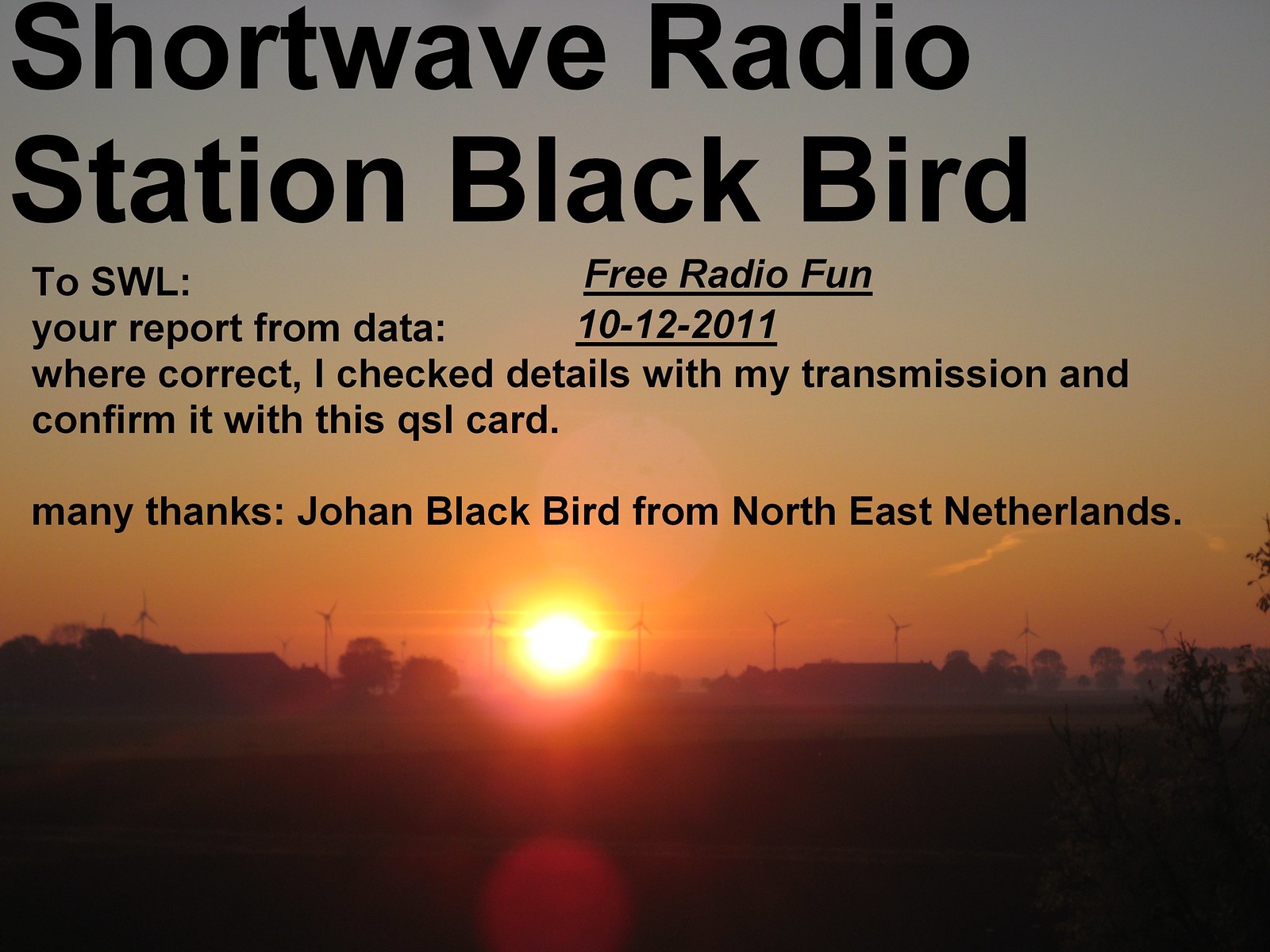This image is a detailed graphic for a shortwave radio station called Blackbird. The background features a picturesque sunset with a spectrum of vibrant colors ranging from orange to light blue, and a visible sun that emits a yellow-gold hue. The scene includes a rural landscape with scattered trees and a field dotted with wind turbines, adding to the serene yet dynamic atmosphere. Superimposed over this sunset are two rows of bold, large black text that read, "Shortwave Radio Station Blackbird." Below this, in slightly smaller text, it says, "To SWL, your report from data were correct. I checked details with my transmission and confirmed it with this QSL card. Many thanks, Johan Blackbird from Northeast Netherlands." Additionally, the image includes italicized and underlined text stating, "Free Radio Fun," with the date "10-12-2011" beneath it. The combination of natural beauty and informative text provides both visual appeal and important broadcast verification.